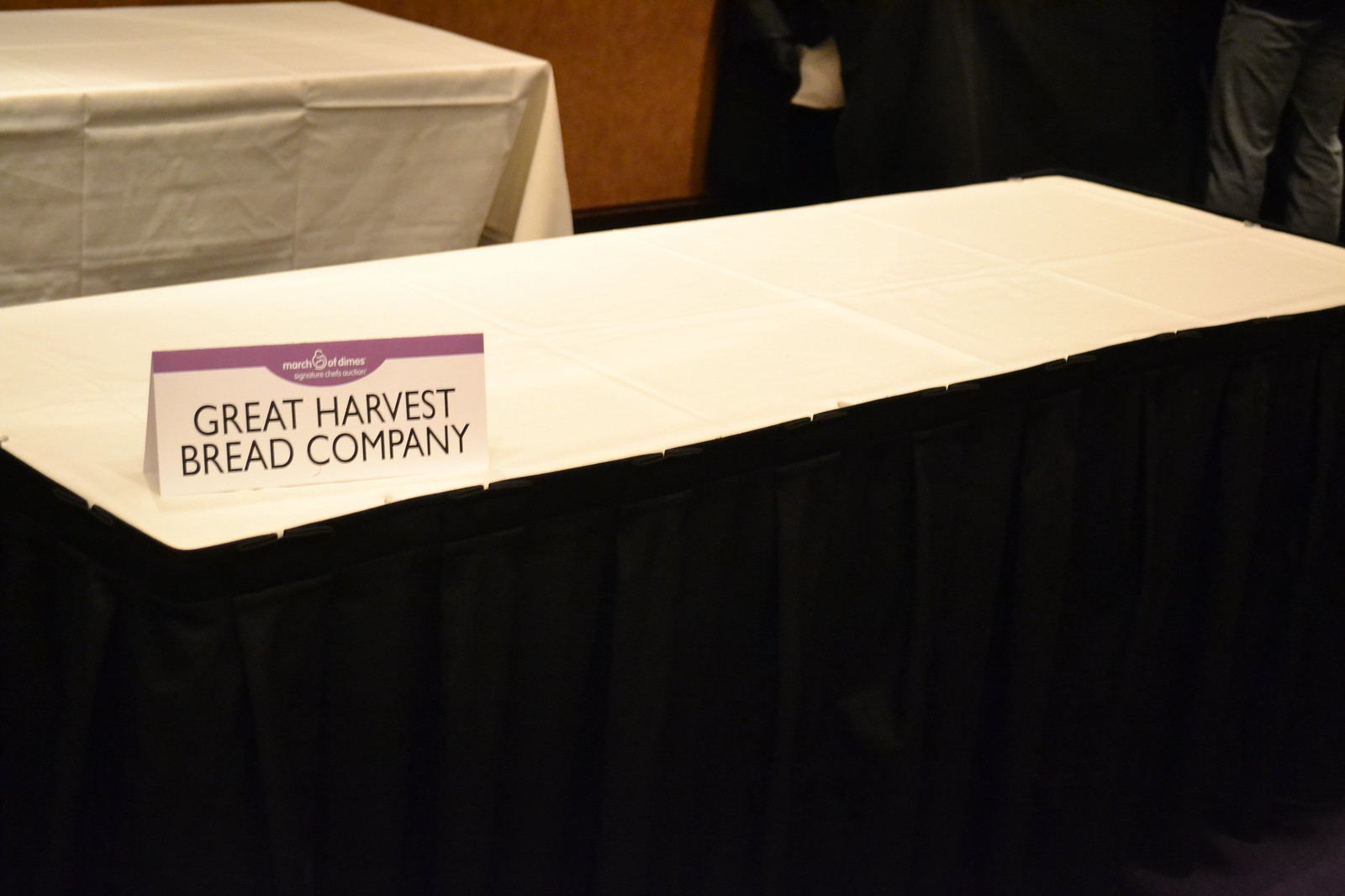The photograph taken indoors showcases two prominent tables arranged against a backdrop. In the foreground, a long rectangular table is covered with a white tablecloth and adorned with a black drape that cascades to the bottom of the image. Positioned on this table is a notable cardboard stand with a white background and a purple top section. The stand prominently displays the text "Great Harvest Bread Company" in bold black letters. In the background, another rectangular table is visible, similarly dressed in a pristine white tablecloth with evident folding creases. Off to the right, a partial view of an individual's lower legs, clad in blue jeans, is noticeable, adding a human element to the otherwise static setting. The upper right corner of the image is further defined by more black drapery, continuing the theme from the foreground table.